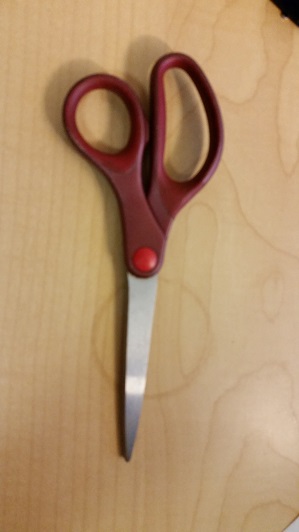The color photograph captures a top-down view of a light brown wooden desktop, prominently featuring a noticeable water stain in the shape of a ring, likely from a glass or can. The wood grain is clearly visible, adding texture to the scene. Centrally placed on the desktop is a pair of full-sized scissors with silver blades. The handles of the scissors are predominantly dark burgundy plastic, with a lighter red color on the inside where the fingers are placed. The pivot point of the scissors is marked by a defined red circle. The positioning of the scissors casts subtle, downward shadows, indicating the overhead angle of the photograph.